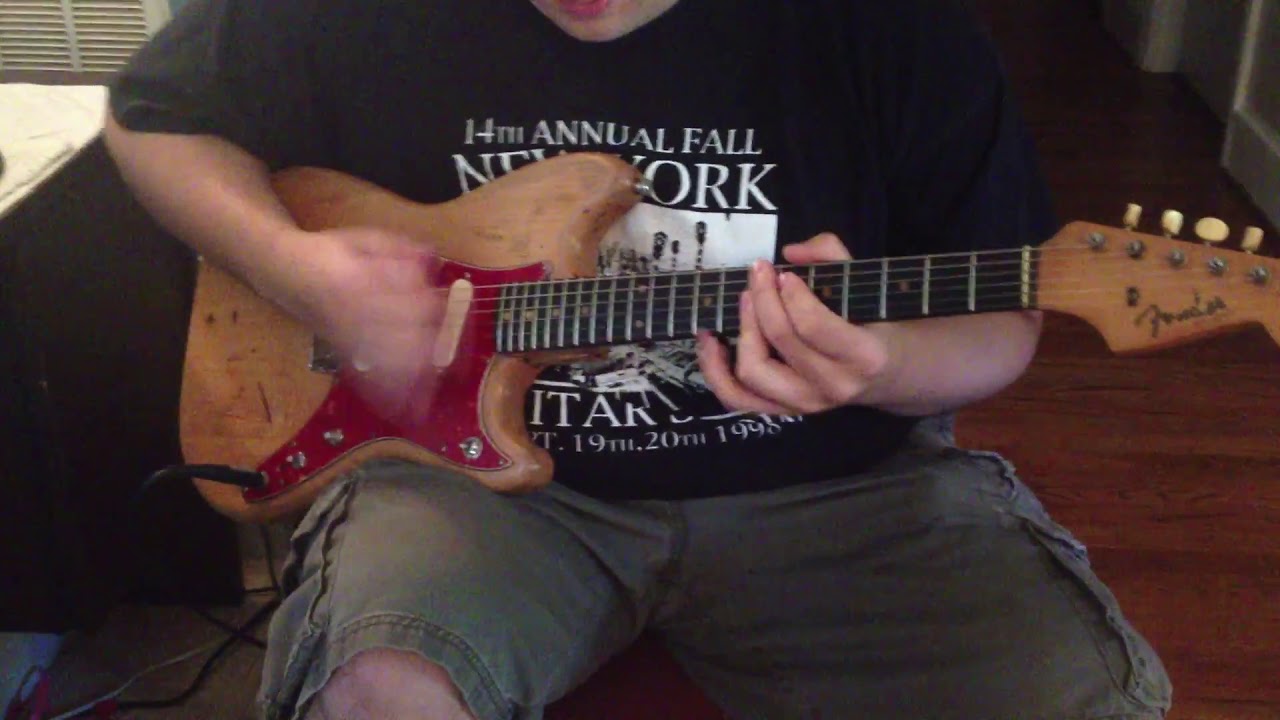The image captures a heavyset individual with a masculine build, seated indoors on what appears to be a hardwood floor. They are playing a Fender electric guitar, characterized by its wooden grain with red detailing, which looks slightly aged with peeling paint. The person is actively strumming the guitar, as evidenced by the blurred motion of their hand. They are wearing a black t-shirt with partially legible text that reads "14th Annual Fall New York" and possibly some additional lines that are not clearly visible. The person is also dressed in dark gray or green shorts. The room is sparse, with a door visible on the left and a desk on the right, subtly suggesting a home environment. A wire connects the guitar to an unseen source, indicating that the instrument is in use.